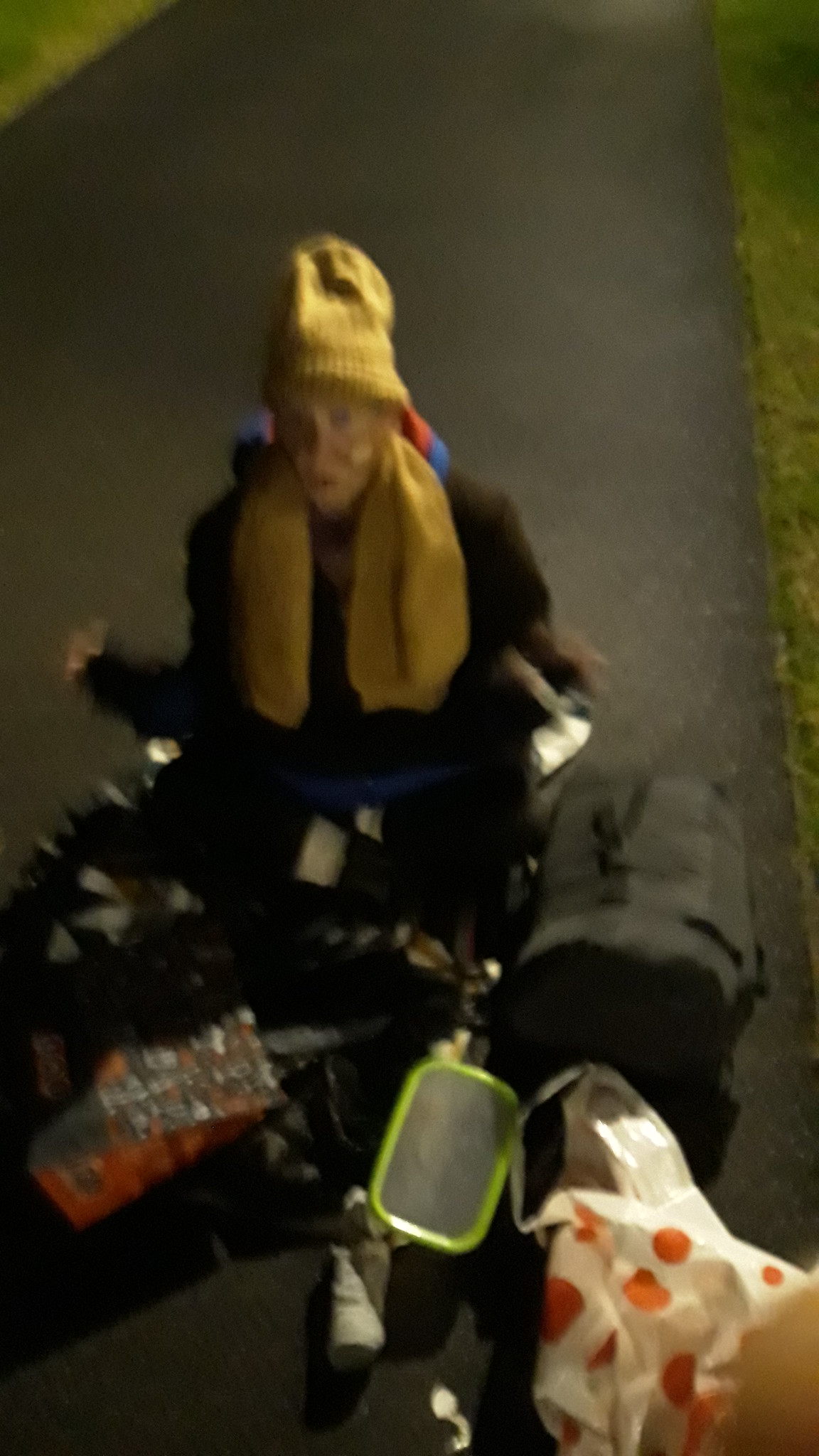This photograph, taken at night from a vehicle, captures a Caucasian homeless individual sitting amidst a clutter of personal belongings in what appears to be a pedestrian walkway. The image, shot in vertical or portrait mode, is rather blurry and out of focus, adding to the somber atmosphere. The subject, who could be male or female, is wearing a dirty, oversized yellow watch cap that extends down to their chest area, resembling ears. A matching yellow scarf, equally worn, wraps around their neck. They are clad in a black coat and seem to be in their older years. Surrounding them are various items, including a black duffel bag, a white bag with red polka dots, and a plastic container, all contributing to the scene of hardship and resilience. The dim street lighting enhances the mood of the photograph, accentuating the stark reality of homelessness.